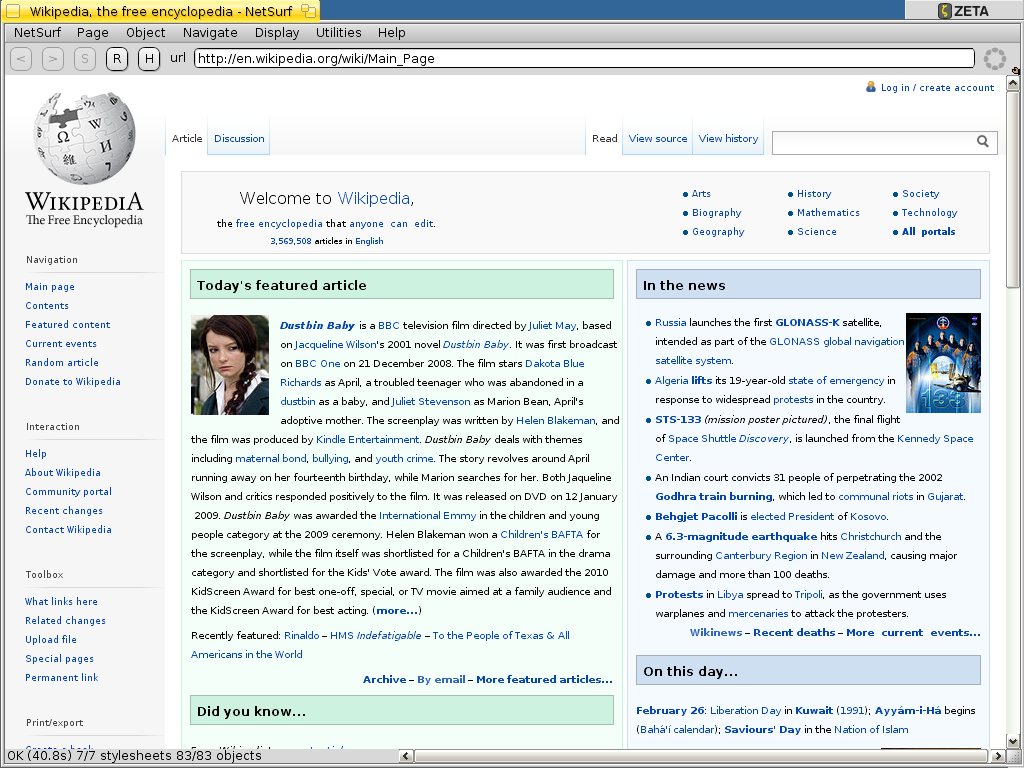**Descriptive Caption:**

The image is a screenshot of a webpage, prominently displaying the header "Wikipedia: The Free Encyclopedia" against a gold background. To the right, the page transitions to a blue section with the word "ZETA" in the upper right corner on a gray background. Below it is a gray navigation bar, listing options such as "Net Surf," "Page," "Object," "Navigate," "Display," "Utilities," and "Help." Further down, another navigation bar features back and forward buttons along with buttons labeled "S," "R," and "H." The URL displayed in the address bar is "http://en.wikipedia.org/wiki/Main_Page."

On the left side of the webpage is the standard Wikipedia navigation menu. Below this, the page's main content begins with the text "Welcome to Wikipedia, the free encyclopedia that anyone can edit," followed by a current count of articles in English, totalling 3,569,508. The section then highlights today's featured article, which is about "Dustbin Baby," a BBC television film directed by Juliet May and based on Jacqueline Wilson's 2001 novel of the same name. The film premiered on BBC One on December 21, 2008, and stars Dakota Blue Richards as April, a troubled teenager who was abandoned in a dustbin as a baby, alongside Juliet Stevenson.